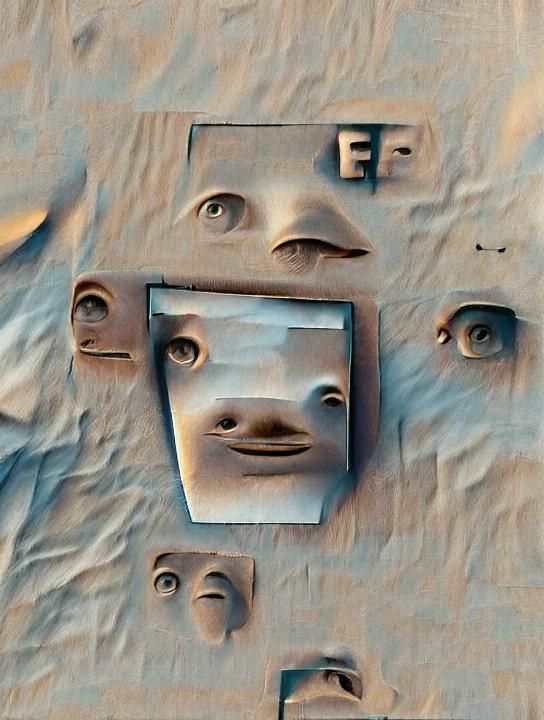The image is an abstract, surreal work of art oriented in portrait mode. Its background, a light to medium brown with wave-like textures, resembles both sand and cloth, enhanced by light and shadow to provide depth and texture. Numerous facial features protrude through torn sections of this background, creating a disjointed and distorted array of eyes, noses, and mouths. Notably, there are two eyes positioned irregularly, a nostril that appears as an eye, and a misshapen mouth. This cacophony of features suggests an abstract face or faces, reminiscent of animals, with textural details such as a furry nose and scattered grains of hair. The colors predominantly include beige and white, with darker brown or black accents, and occasional streaks of blue and orange. The image gives an AI-generated impression due to its blurriness and washed-out quality. There is a vague semblance of text near the top that could be interpreted as "FP," although it appears incidental.